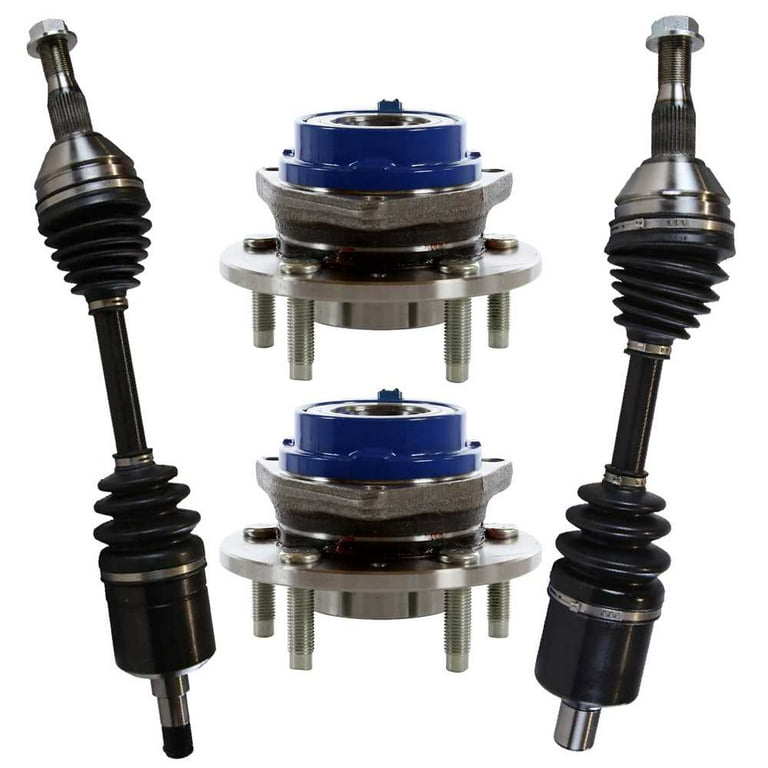This photographic image, set against a white background, depicts industrial automotive equipment. There are four distinct pieces, each mirrored on either side of the frame. To the left and right are vertical assemblies featuring silver pistons at their base, followed by alternating black cylinders and bellows, topped with tapered cylinders crowned by lid-like caps. In the center, two identical blue and silver components sit on four metal legs each, resembling intricate machinery possibly described as "core generator starter accelerator flux capacitors." These central pieces are composed of multiple detailed elements, including a cylindrical blue body, gray gaskets, and a tiered silver structure. There is no accompanying text in the image.